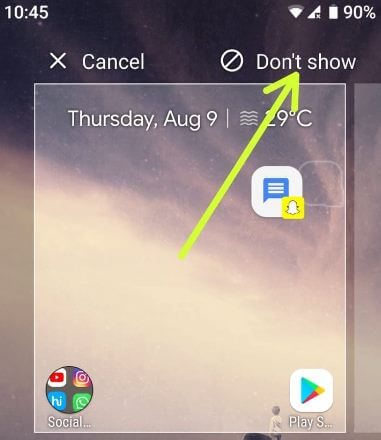The image is a detailed screenshot from a smartphone interface, captured at 10:45. In the top-left corner, the time is displayed, while the top-right corner shows a nearly complete WiFi signal and a battery level at 90%. Below these indicators is an interface containing an 'X' button labeled 'Cancel,' adjacent to a 'Don't Show' option symbolized by a circle with a diagonal line. Highlighting this option is a yellow arrow pointing towards the word 'Don't.'

The background of the image features a gradient that transitions from black at the top, through purple, and then to a gray hue at the bottom, giving an impression reminiscent of blurry clouds in the sky. Dominating the center is a rectangular box with a gray border, displaying the date "Thursday, October 9" and the temperature "29 degrees Celsius." Inside this box, there's another small text box with an ellipsis ("...") in the middle and a Snapchat icon within the same frame. Finally, the Google Play Store logo is positioned in the bottom right corner of the image.